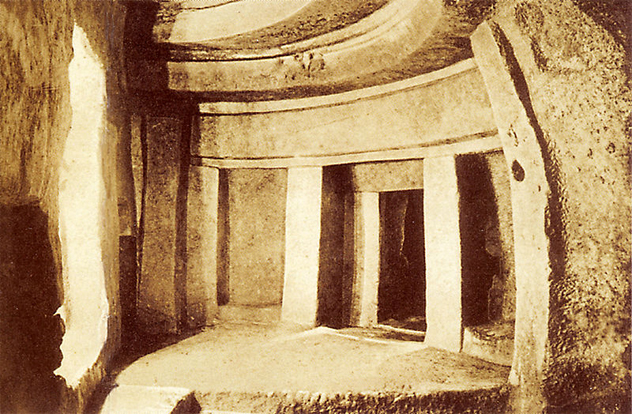The image depicts an ancient, sepia-toned scene dominated by intricately carved stone ruins built into a rock face. Centered within the rectangular frame, which is wider than it is tall, stands a grand doorway flanked by two light-hued columns, in stark contrast to the dark brown shadows cast upon them. Above these columns stretches a smooth, horizontal stone lintel, giving the entrance a stately appearance. On the right side of this doorway, the rock surface varies from a nearly smooth, curved area to rough, jagged textures, suggesting the natural rock formation surrounding the carved structure.

The left side of the image reveals a mysterious, elongated bright area with jagged edges that extends almost from the top to the bottom of the frame, potentially an opening letting in light. The entirety of the structure seems to curve inward, resembling an inner chamber or room hewn directly from the stone, complete with squared lintels and rectangular cut-outs that might serve as windows or additional doorways. The ground in front of the doorway forms a triangular platform that tapers off and disappears into darker shadows, hinting at steps or a drop-off, though its exact nature is obscured.

Overall, the scene is bathed in a dark tan, sepia hue, lending an ancient and timeless quality to the stone architecture, which conveys a sense of mysterious antiquity and skilled craftsmanship.